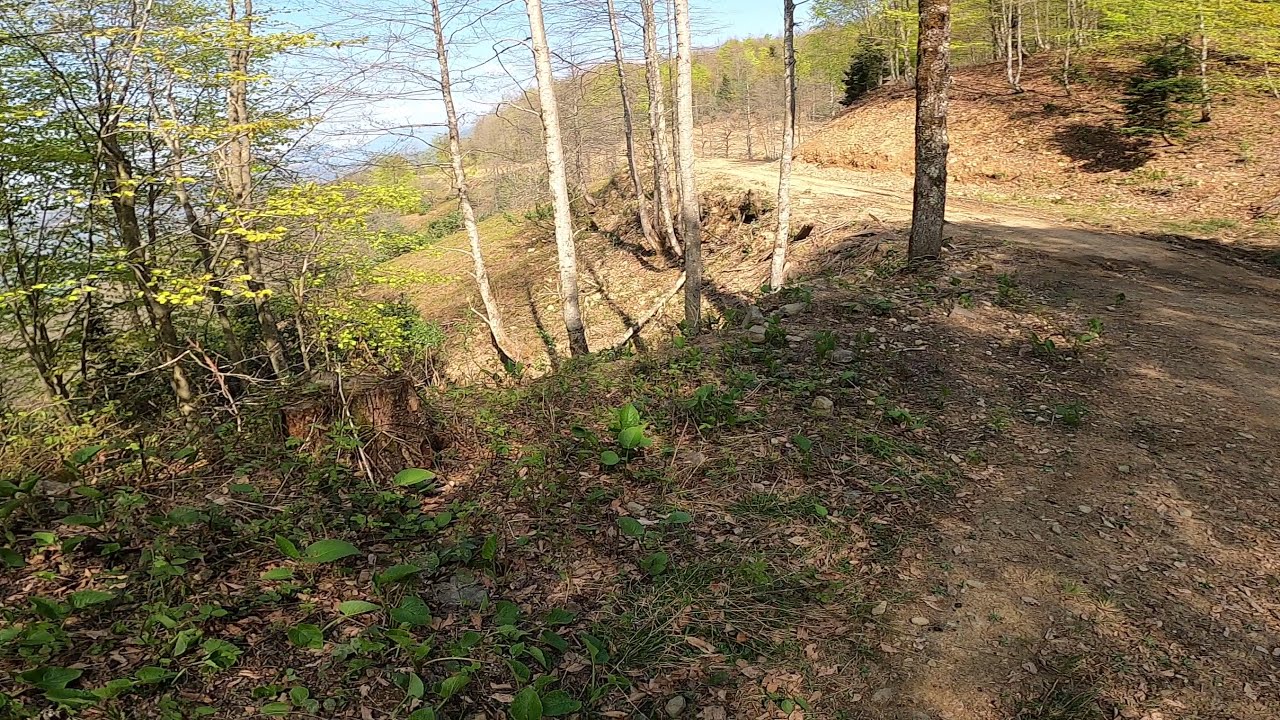The image captures a horizontally aligned rectangular scene of a serene, forested area bisected by a compacted dirt road. Running through the center and extending towards the right, this narrow trail invites the eye to journey through a landscape adorned with diverse trees and vegetation. On the right side, the terrain rises slightly with an incline dotted by a few trees, their sparse foliage creating an airy canopy. Centered in the frame are trees with light gray trunks, their branches bare and stark against the sky, contrasting with the vibrant green and yellow leaves on the trees to the left. The top left corner reveals a clear blue sky adorned with feathery white clouds, while distant mountains add depth to the background. The forest extends endlessly, with leaves and branches scattered across the ground, mingled with rocks and new growth peeking through. This meticulous composition showcases nature's tranquil beauty and seasonal transition.